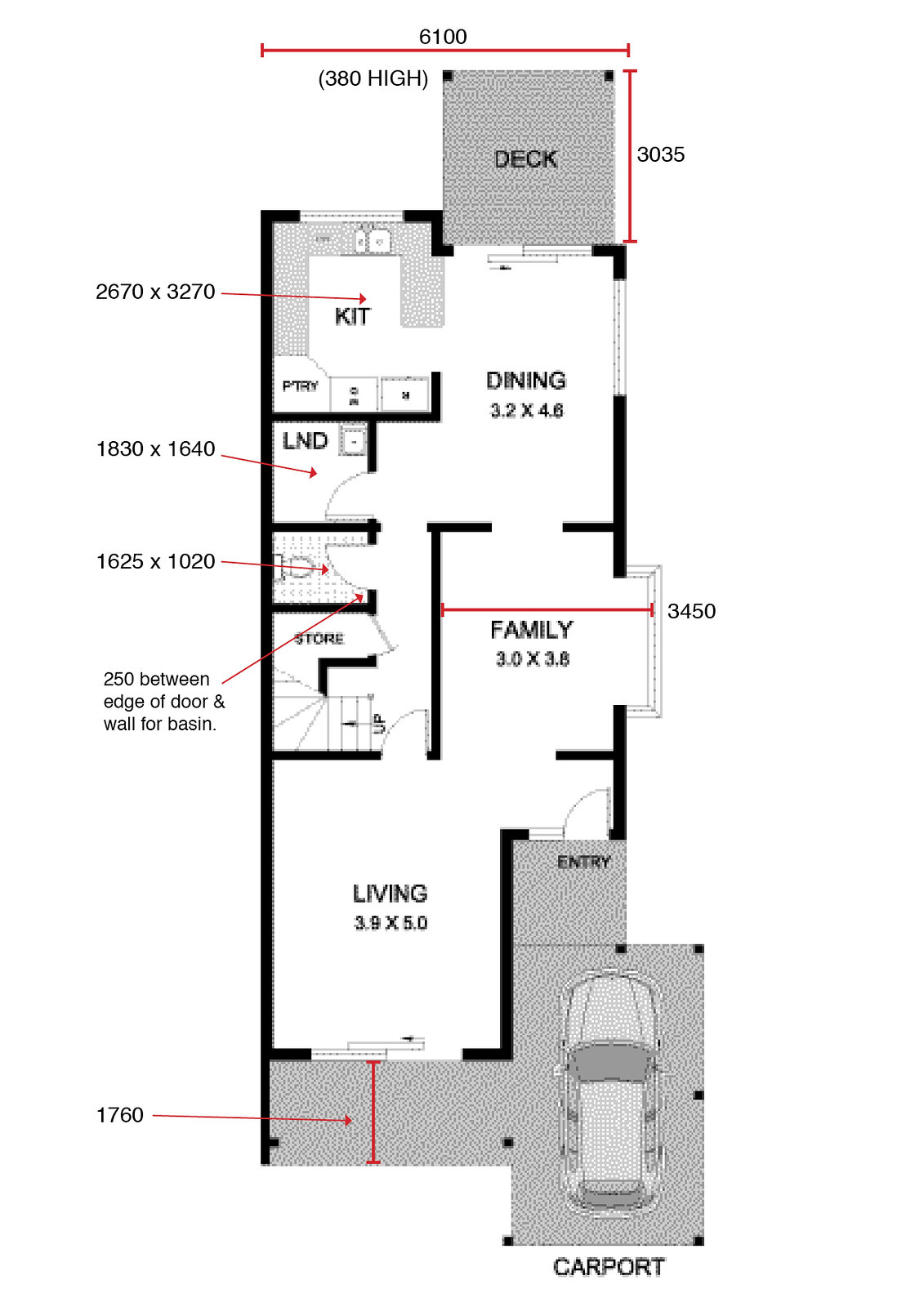This detailed caption describes a complex layout, presumably of a house or apartment, showcasing various dimensions and labels:

---

The image displays a detailed layout of a residential space, possibly a house or apartment. At the top of the layout, there's a gray square labeled "deck" in black, featuring two black boxes—one in the upper left and one in the upper right. The left side is annotated with "380 high" in parentheses. A red horizontal line runs across the deck, marked with "6,100" in black, and another red vertical line on the side indicates "3,035."

Below the deck, the plan transitions into a primarily rectangular shape. The "dining" area is labeled in black on a white background, and its dimensions are provided as "3.2 by 4.6." Beneath the dining area, there's a section labeled "family," also on a white background, with dimensions that are partially obscured but likely "3.0 by 3.6" or "3.8."

At the bottom of the structure is a gray box labeled "entry" in black. Adjacent to it is another gray box containing a car graphic and labeled "carport" in black. To the right of the carport, a red line is annotated with "1,760" in black.

The "living room" is positioned above the carport and dining area, labeled in black on a white background with dimensions "3.9 by 5.0." Above the living room, there are stairs labeled "up" and a smaller area noted as "store." On the left side of the stairs, a note in black indicates "250 between edge of door and Waffle Basin."

To the right of the living room, there is a "bathroom" labeled with a red arrow and dimensions "1,625 by 1,020" in black. Above the bathroom, a space is labeled "L and D" (potentially "Laundry and Drying") with dimensions "1,830 by 1,640." Adjacent to this, the "kitchen" (abbreviated as "kit") is outlined with a red line and the dimensions "2,670 by 3,270" in black.

---

This revised caption meticulously details the layout’s components, providing a clear and structured description of each section’s location and dimensions.